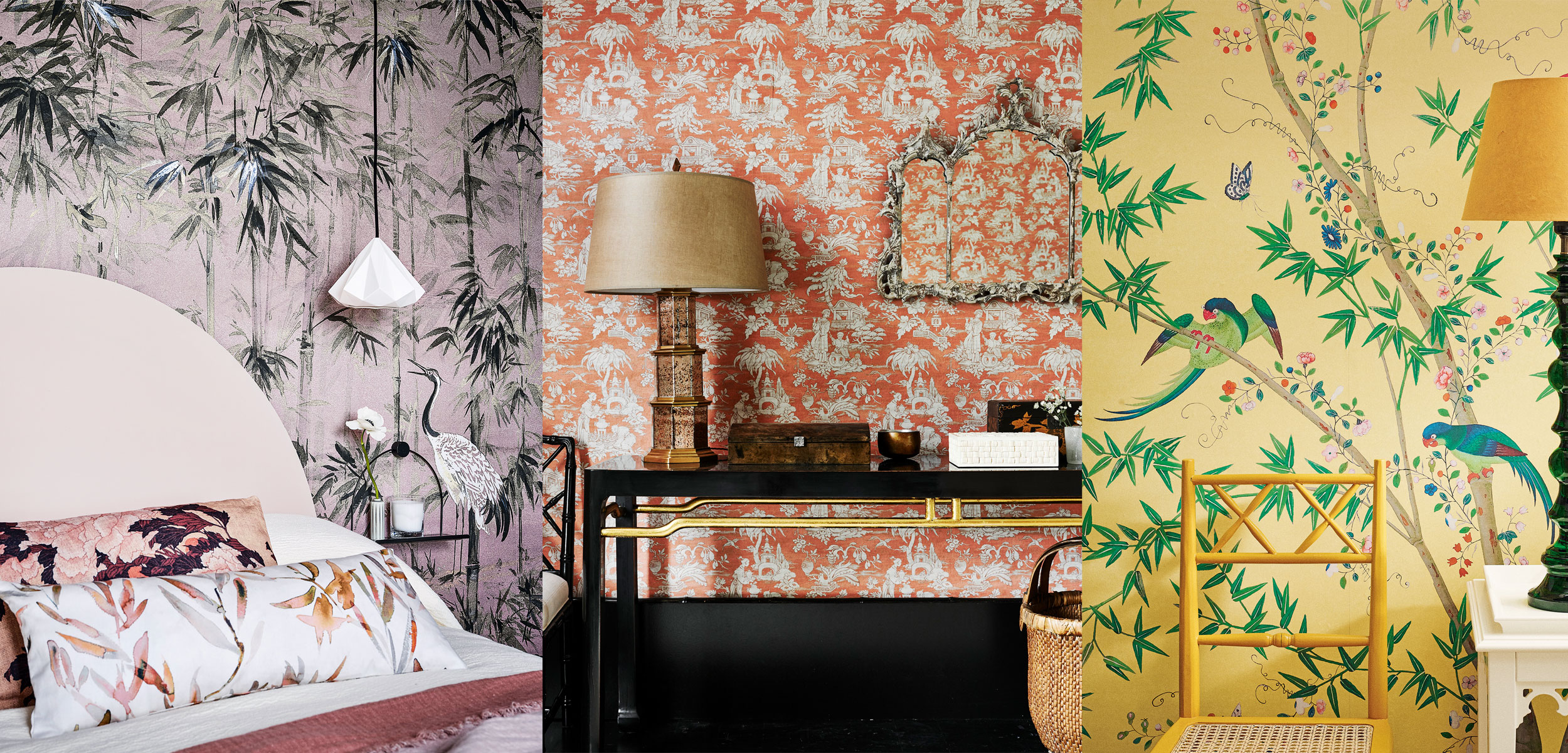This composite photograph presents three distinct interior settings, each showcasing unique and vibrant wallpaper designs. The image on the left features a bedroom adorned with bamboo-themed wallpaper accompanied by a hanging ceiling light. The bed sports a grand, round headboard and is complemented by two long body pillows encased in bamboo chute-printed pillowcases. The center image depicts a dining room characterized by its intricate orange and white wallpaper with tropical tree motifs; a black table with gold trim dominates the scene, topped with a stylish lamp and other decorative items. The right-hand image highlights a room with wallpaper rich in botanical themes, featuring tropical trees with perched birds, a yellow wicker chair, a white table, and a lamp with a dark wooden base and a coordinating lampshade.